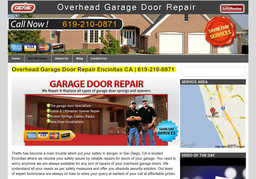The top section of the image features a long gray rectangle with white text that reads "Overhead Garage Door Repair." Below this, there is an image of a brick home characterized by a triangular gable roof. The front of the home showcases two garage doors, a large white window, and a white entrance door. 

Inside a black rectangle overlaying the image, the text "Call Now 619-210-0871" appears in yellow font. The graphic also displays icons representing accepted credit cards: American Express, Visa, and MasterCard.

Towards the bottom, a yellow rectangle contains the text "Overhead Garage Door Repair Encinitas, CA," along with the repeated phone number "619-210-0871." 

Additionally, the image includes a photo of two men dressed in black polo shirts, baseball hats, jeans, and equipped with tool belts. They are standing in front of another home with primarily brown exterior.